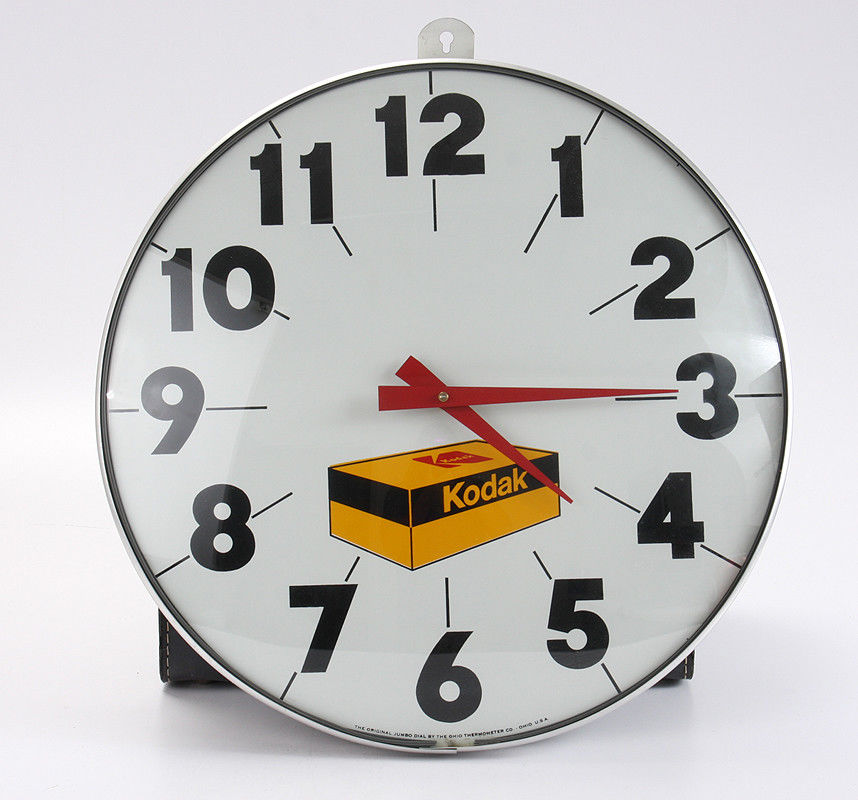The image is a detailed advertising photo of a large, photorealistic, round wall clock set against a white background. The clock face is white with bold black numerals arranged in a typical 12-hour format. Each numeral is accompanied by a small line above and below it as part of the design. The outer rim of the clock is black, adding a crisp contrast to the face. At the top of the clock, a small plastic loop with a keyhole cutout allows it to be hung on a wall. The clock displays the time of 4:15 with elongated, pointed red hour and minute hands connected at the center by a small silver screw. Below the center of the clock, almost directly above the number 6, is a color illustration of a Kodak film box. The classic Kodak branding features a yellow rectangular box outlined in black, with "Kodak" written in a bold font and a red insignia at the top. The entire clock is propped against a black leather base.